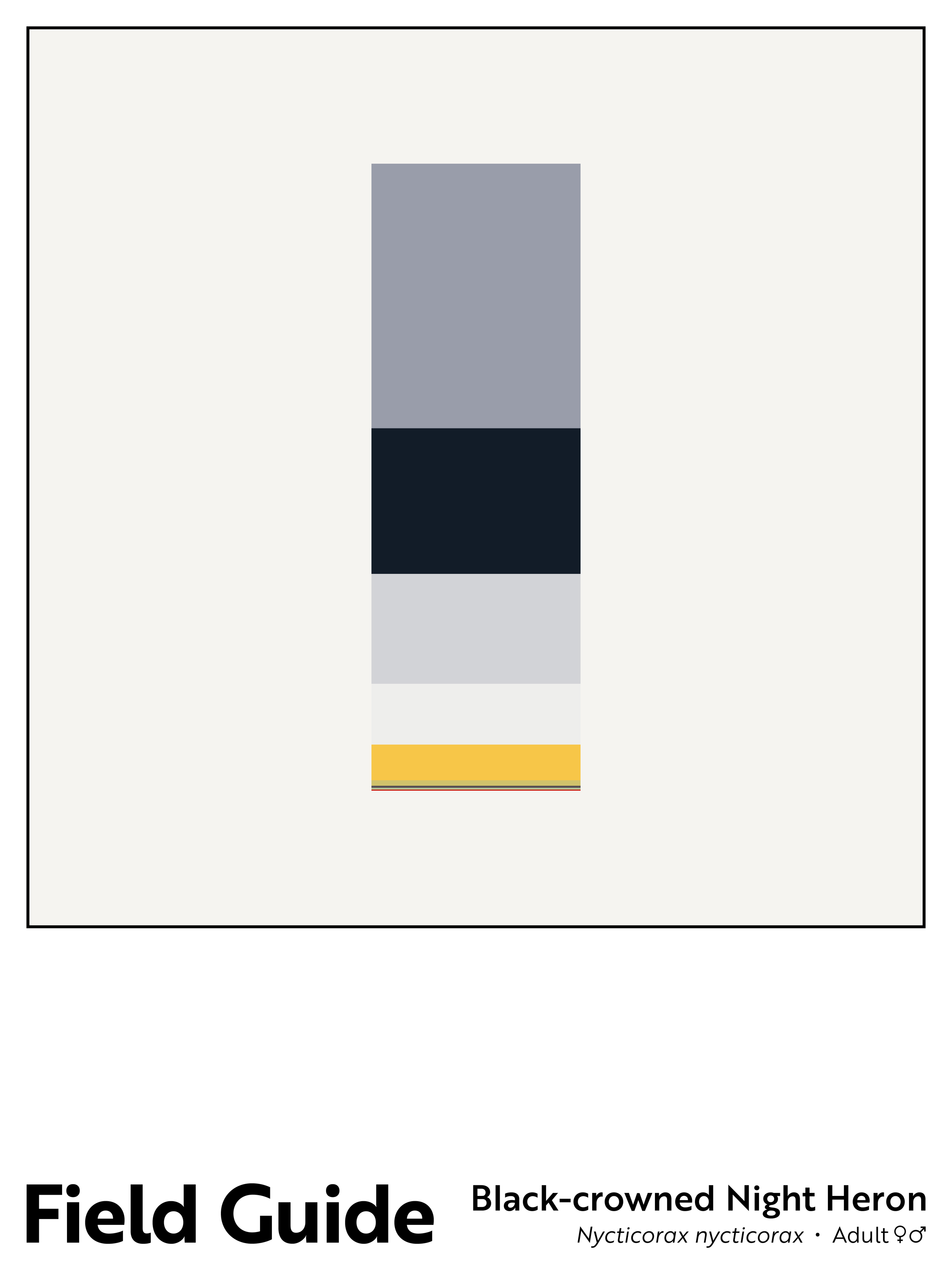The image features an abstract illustration occupying the upper half, set against a beige background with a black outline. The composition consists of a vertical column of solid-colored rectangles, which progressively decrease in size. Starting from the top, a large gray rectangle is followed by a slightly smaller black rectangle. Below it, a light gray rectangle appears, about 70% the size of the black one. This is followed by a white rectangle, approximately half the size of the light gray one, and then a yellow rectangle, 70% the size of the white one. As the sequence continues, the rectangles become increasingly diminutive, resembling lines, with a green one followed by a blue one and finally a red one.

Below the illustration, a section of text reads "Field Guide: Black Crowned Night Heron, Nyctocorax nyctocorax, adult male, female." This caption, presented in large text (but not all caps), provides a scientific context, seemingly unrelated to the abstract art above. The entire design creates a juxtaposition of artistic abstraction with scientific labeling, framed within a visually distinct, bordered format.